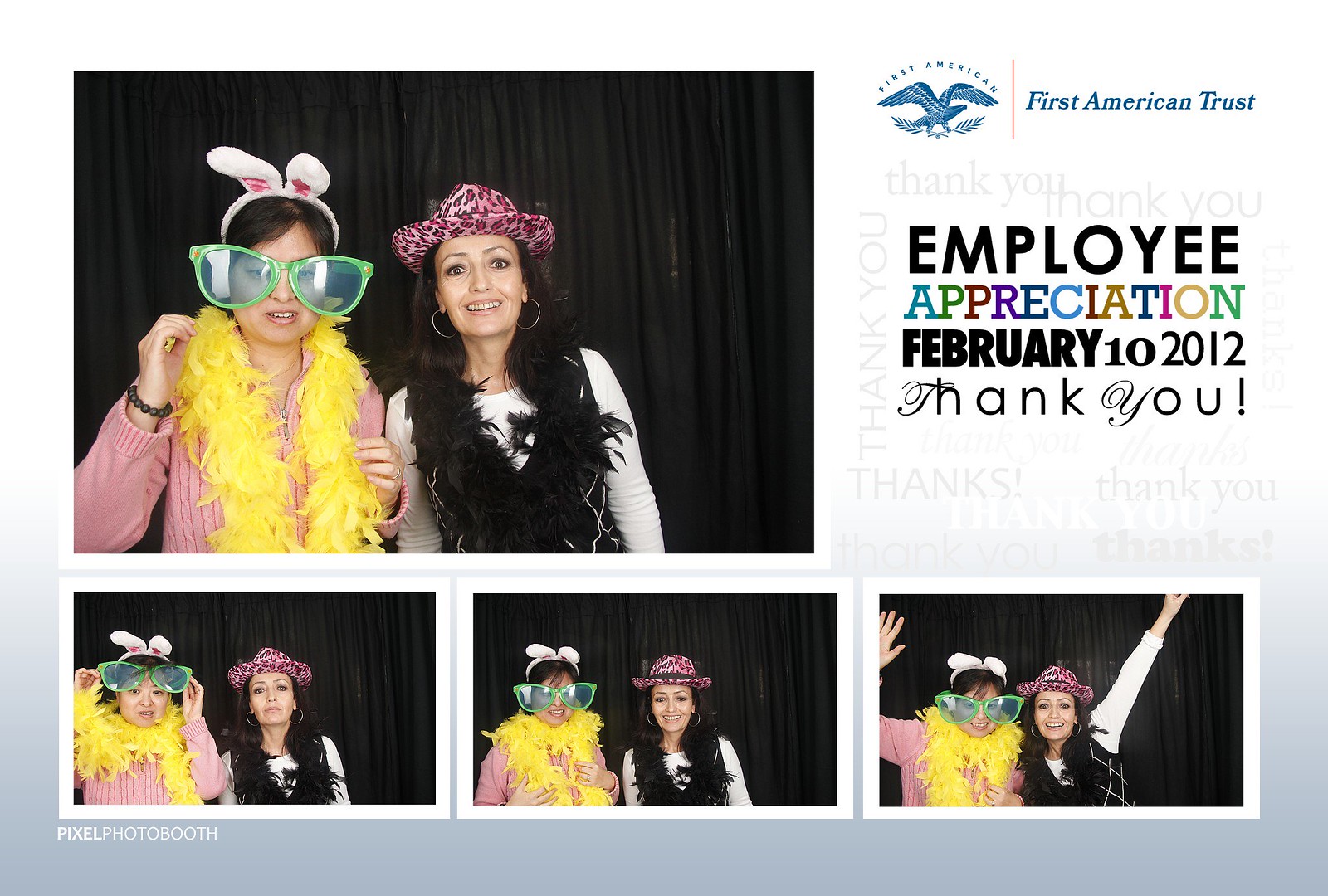This image appears to be a postcard featuring a collection of four photographs, showcasing two women using playful props, likely taken at an event photo booth during an Employee Appreciation event for First American Trust on February 10th, 2012—according to the text and logo positioned at the top right corner. The largest photo is located at the top left, displaying the women standing side by side, looking directly at the camera.

The woman on the left is adorned with oversized green sunglasses, bunny ears, a yellow feather boa, and a pink sweater. Her companion on the right sports a pink and black leopard print cowboy hat, hoop earrings, and a black feather boa over a white long-sleeve shirt. Both women exude a playful and festive vibe, further highlighted by their contrasting but brightly colored accessories.

Beneath this principal image, there are three smaller photographs arranged horizontally. Each one captures the same women in slightly different poses but still with their distinct accessories. The colors present in the image include blue, white, black, green, purple, tan, brown, and a notable extent of pink, tying the photos together visually within a gray and white bordered background. The dynamic layout and joyful expressions illustrate a lively and memorable moment from the event.